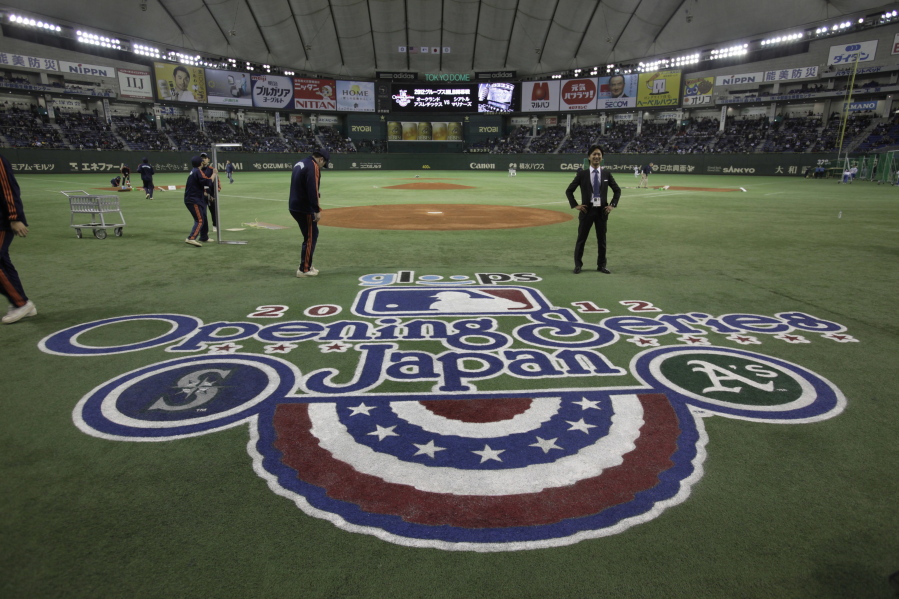This detailed photograph captures an indoor baseball stadium in Japan, specifically the Tokyo Dome. The field is predominantly grass with dirt areas at each base, diverging from the typical all-dirt diamond. Centered prominently on the turf is a large, colorful logo with bunting painted in red, white, and blue stripes and stars. The logo reads "2012 Opening Series Japan," with the Major League Baseball logo featuring a player hitting a ball. In the stadium, a man in a suit and blue tie stands with his hands on his hips in the middle of the grassy area, while workers in track suits can be seen setting up the field. The packed audience is seated around in the stalls, creating a lively atmosphere. Surrounding the stadium's perimeter, Japanese advertising billboards are visible. Above an electronic screen playing ads, "Tokyo Dome" is prominently displayed. The enclosed stadium also features skylights where the walls meet the roof, allowing natural light to filter in.